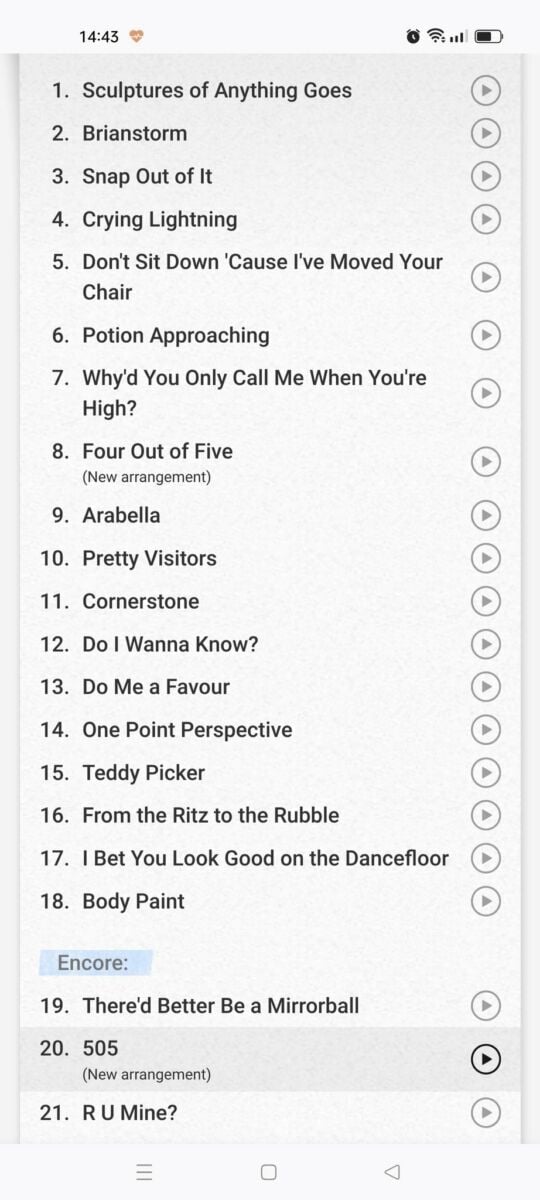A digital screenshot featuring a white background and a list of eighteen items. Each item in the list is accompanied by a circular play button symbol, represented by a triangle within a circle, positioned to the right of the item. The list is structured numerically as follows: 

1. **Sculptures of Anything Goes**
2. **Brainstorm**
3. **Snap Out of It**
4. **Crying Lightning**
5. **Don't Sit Down 'Cause I've Moved Your Chair**
6. **Potion Approaching**
7. **Why'd You Only Call Me When You're High?**
8. **Four Out of Five** _(New Arrangement)_
9. **Arabella**
10. **Pretty Visitors**
11. **Cornerstone**
12. **Do I Wanna Know?**
13. **Do Me a Favour**
14. **One Point Perspective**
15. **Teddy Picker**
16. **From the Ritz to the Rubble**
17. **I Bet You Look Good on the Dancefloor**
18. **Body Paint**

At the bottom of the list, there is a blue rectangle with the word "Encore" inscribed within it.